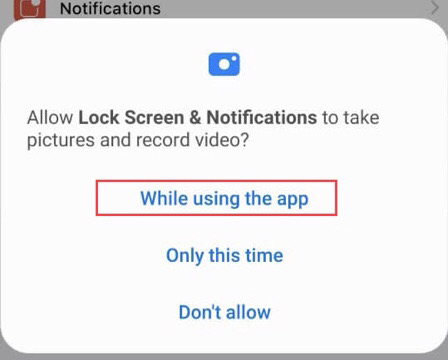The image is a screenshot of a notification prompt with a rounded-square shape. The main notification area has a white background, bordered by gray at the top and bottom edges, indicating an overlay effect. At the top of the notification is a small blue camera icon encased in a white circle, with another tiny white circle on its right side. 

Directly below the icon, bold black text reads: "Allow Lock Screen & Notifications to take pictures and record video." The options for responding are listed beneath in blue text: "While using the app," "Only this time," and "Don't allow." The "While using the app" option is highlighted within a red box.

In the gray background area at the top, the word "Notifications" is visible, accompanied by a red square icon with a white square inside it and a white dot on its top right corner. The overall effect is that the notification prompt visually stands out against the subtly gray, dimmed background.